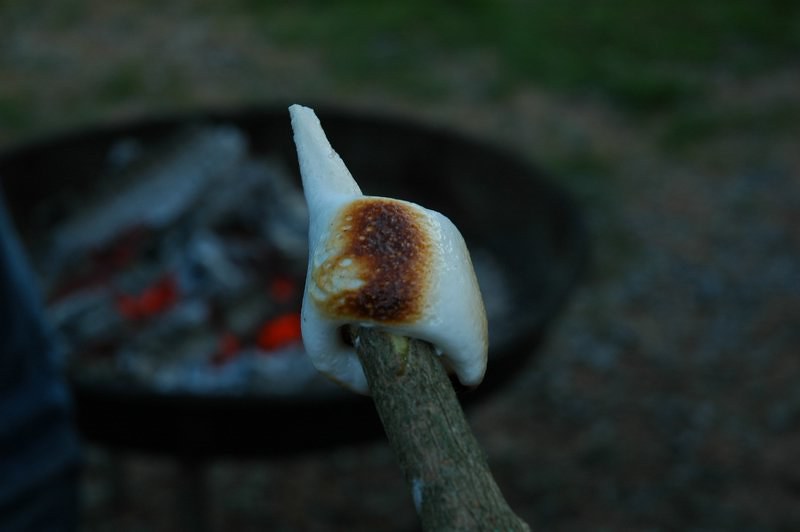The image depicts a first-person perspective of a melting marshmallow on a thick stick, held over a campfire. The marshmallow is adorned with burn marks and is drooping due to its melted state. The stick, which pierces through the bottom of the marshmallow, extends slightly through the top and is enveloped in gooey, white marshmallow. In the blurred background, a barbecue pit filled with burning charcoal and whitish debris fuels the fire, surrounded by a gravelly rock area. The setting also features hints of brown earth and green grass on the right side, suggesting a campground environment. The predominant colors in the image are orange, black, white, brown, green, red, tan, and gray.